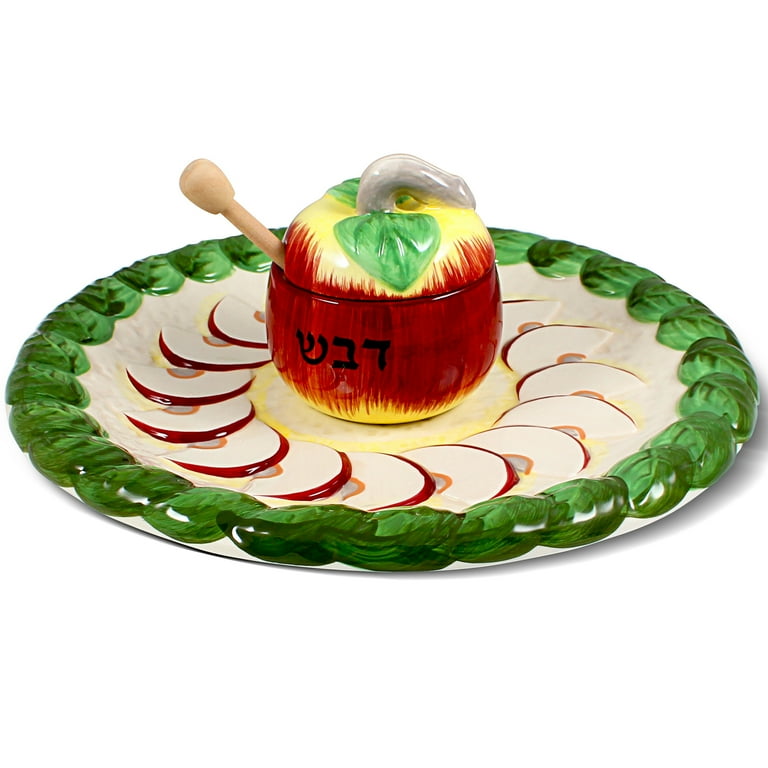The image showcases an intricately designed ceramic serving plate with a central honey dispensing apple-shaped bowl. The round, white plate features an edge adorned with a repeating leaf motif, each leaf overlapping the next. Just inside the rim, a circle of overlapping apple slices is painted, creating a vibrant, decorative border. The centerpiece of the plate is a ceramic bowl designed to resemble an apple. This bowl has a red body with a yellow top, green leaves, and a small white handle resembling an apple stem. The apple-shaped bowl lid matches the bowl's design, and a wooden honey spoon protrudes from its side. This detailed and thematic plate is perfect for serving honey, fruit, and dips, making it an ideal centerpiece for a party or a decorative online advertisement.